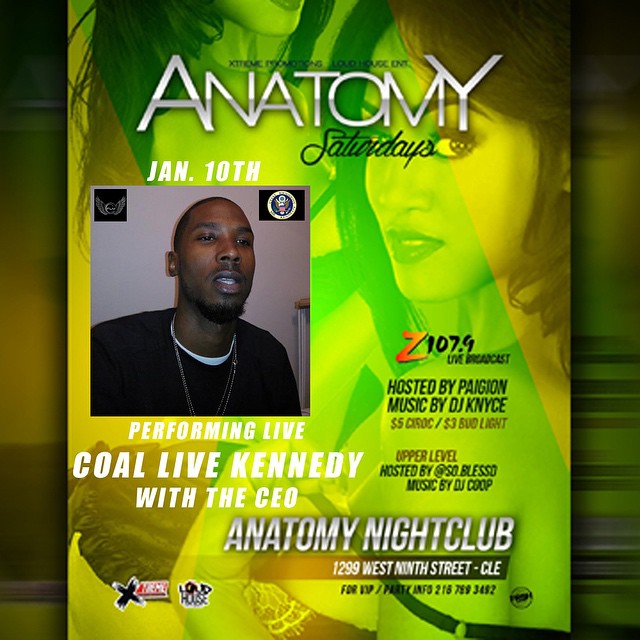This image appears to be an advertisement flyer for an event titled "Anatomy Saturday," scheduled for January 10th. The background is predominantly green with yellow highlights, giving a vibrant and energetic aesthetic. Featured prominently on the flyer is a photograph of a man wearing a black shirt with a white undershirt and chain necklaces, looking to his left. Above this image, text details performances by artist QoLiveKenneth and the CEO. The event is hosted by Paragon Music, with music by DJ Kainais. Additional information includes "Z107.9 Live Broadcast" and promotions such as "$5 Ciroc" and "$3 Bud Light." The address for Anatomy Night Club, 1299 West 9th Street, CLE, along with other logos, are positioned below the main text. In the background image, there are two women wearing short dresses, adding to the flyer’s nightclub theme.